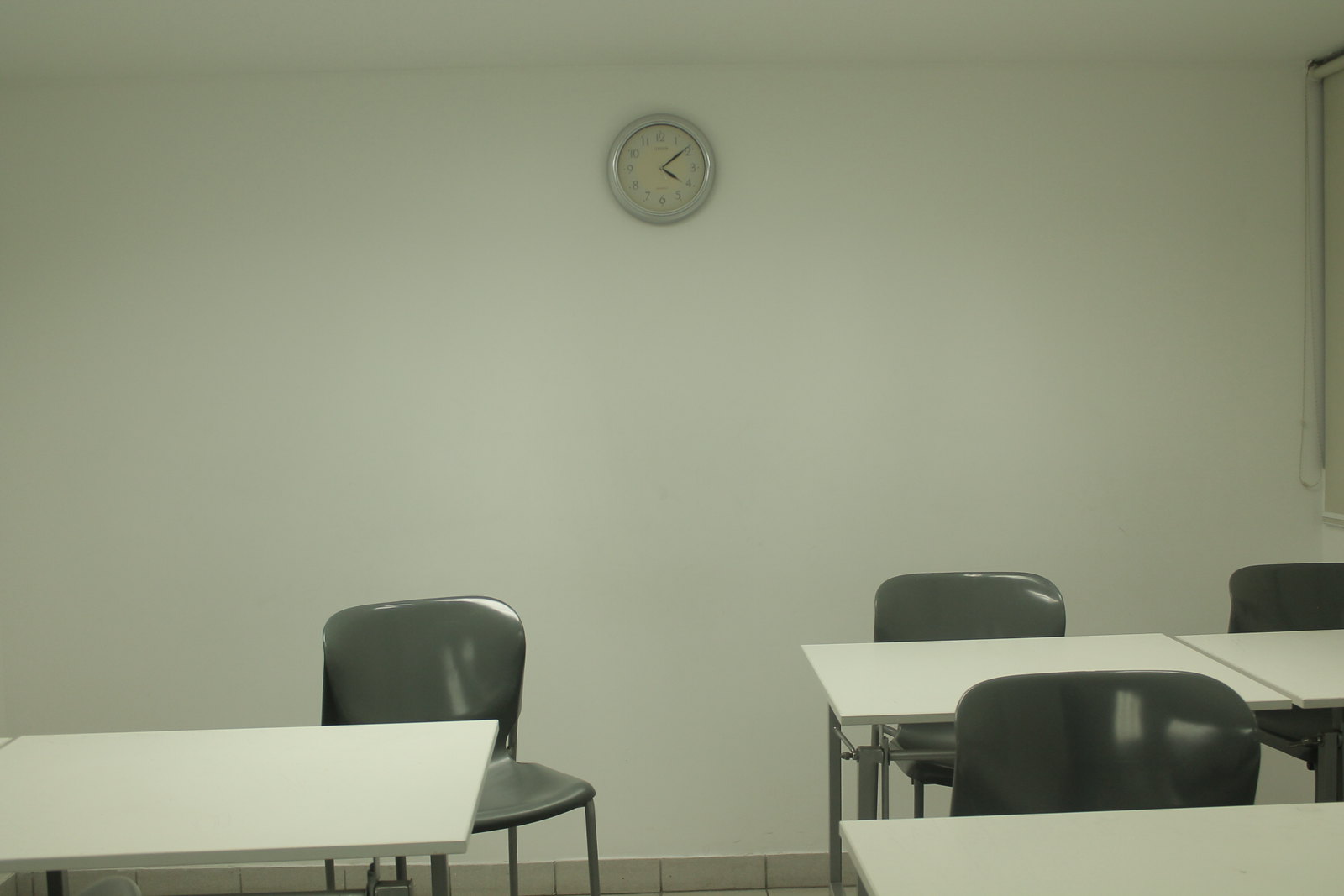This photo depicts a classroom with white walls and ceiling, accented by a gray tile baseboard. The floor is tiled, and the room is equipped with long, rectangular white tables with metal legs, some of which are pushed together to form a longer surface. Scattered around these tables are at least four gray, shiny plastic chairs, though there might be a mix of blue chairs as well. One gray chair on the left is notably crooked, suggesting it was recently occupied. On the back wall opposite the viewer, a silver-framed analog clock with black hour and minute hands reads 4:10. The room lacks any notable decorative elements, presenting a plain, utilitarian ambiance often found in educational settings.